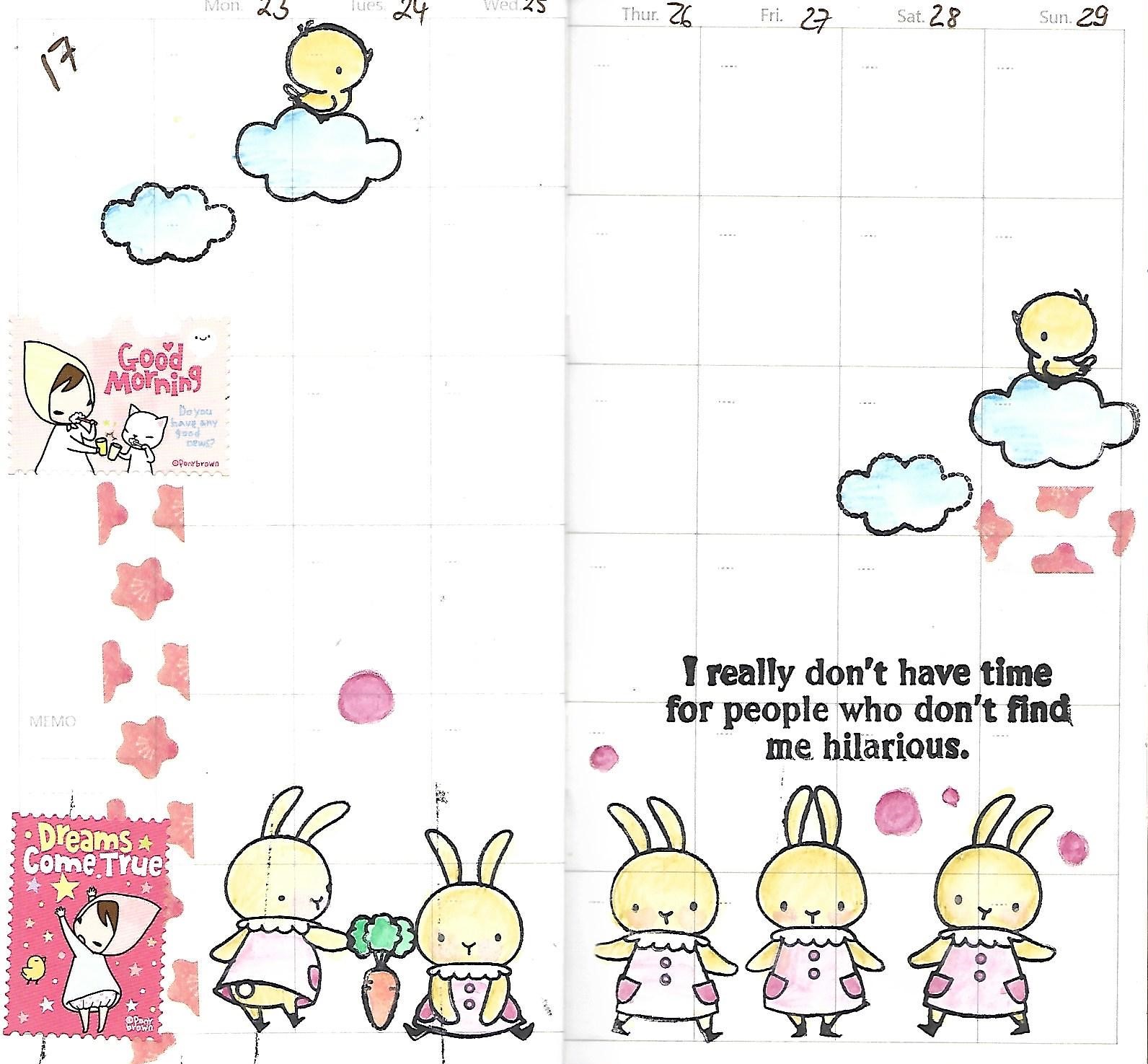This image portrays a whimsical children's calendar featuring a playful assortment of hand-drawn and stamped illustrations. The calendar highlights a week from Monday the 23rd to Sunday the 29th, with the days slightly cut off at the top. Each day's number is annotated by hand, with the number 17 written above them in a European style with a dash through it. The calendar grid is laid out with faint gray lines on a white background.

Adorning the calendar are several charming visuals: two yellow baby chicks ride on light blue clouds, one in the upper left and another in the middle right with an empty cloud beside it. There is a humorous and light-hearted quote at the top that reads, "I really don't have time for people who don't find me hilarious." Alongside these illustrations, a little girl with brown bangs, wearing a kerchief hood, appears in different settings. One stamp shows her toasting a small white cat with the greeting "good morning," while another displays her holding up a star next to a chick with the encouraging phrase "dreams come true," marked in a pink stamp at the bottom left.

Additionally, a series of rabbits dressed in frilly pink dresses with pockets and collars parade across the bottom of the calendar. The depictions vary: one rabbit offers a carrot, another is sitting, while the remaining are either standing or walking—one mirrored from a previous stance. The overall aesthetic is designed for children or those with a whimsical, youthful sense of humor.